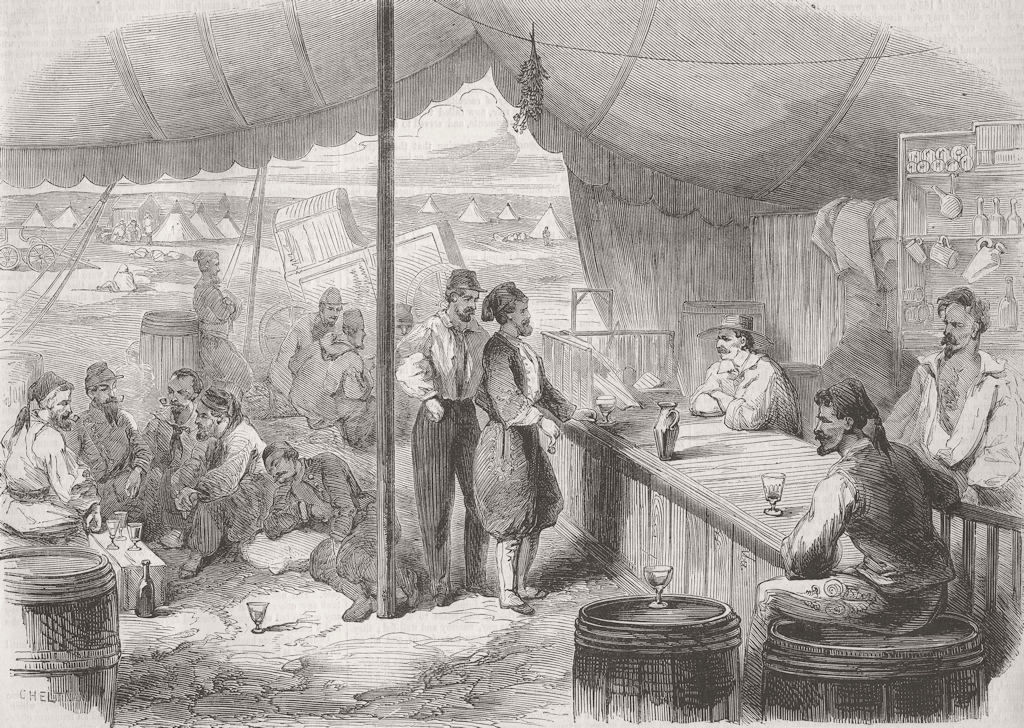The black and white hand-drawn sketch, created with intricate pen and ink hatching, depicts a bustling bar scene set in an Asian or Turkish area. The bar, supported by a central circular post, sits under a tented roof held up by visible ropes. The bar itself is made of wood, and behind it are shelves stocked with various jugs and glasses. 

Two bartenders work in the scene: one, with broad flat-topped hat, leans on his elbows, while the other, sporting a loose white shirt open to his navel, has dark hair, a mustache, and a pointed beard. At the bar, a man in a vest, white shirt, and light-colored pants sits on a wooden barrel, his long hair tied in a tail. He is absorbed with a glass in front of him.

To the right, two patrons stand at the bar; one wears old-style balloon Turkish pants, and the other a peaked cap and striped trousers. On the ground near them are five more men, either sitting or kneeling on blankets, engaged in conversation or a game. Their drinks rest on the ground or a small footstool beside them. The background reveals more tents and faintly sketched clouds, adding depth to the lively, nostalgic atmosphere.